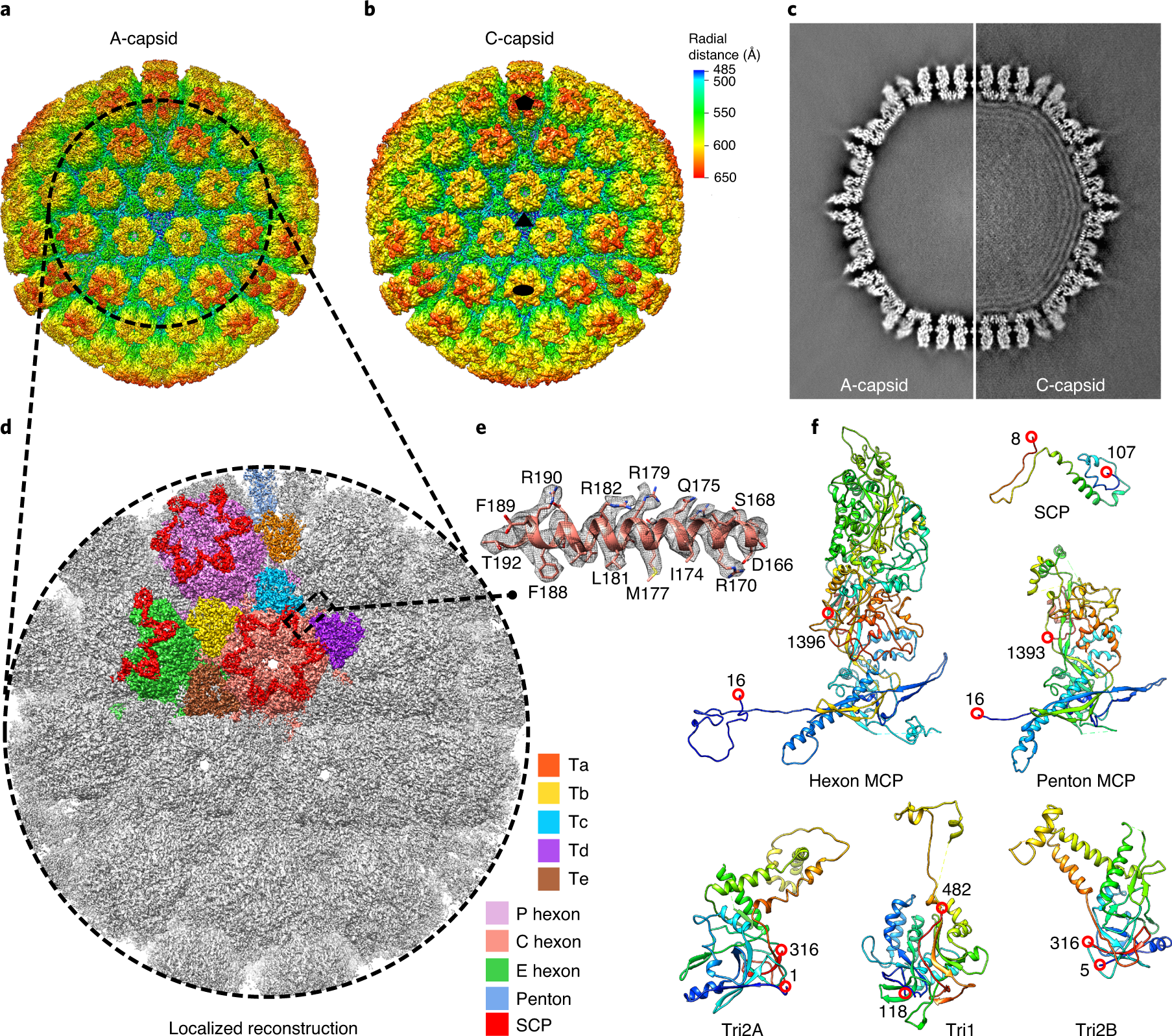This image is a detailed scientific illustration focusing on the structural and infrared analysis of capsids, specifically A capsid and C capsid. The upper left corner features two small green circles labeled as A capsid (A) and C capsid (B), with minute spongy areas circled in orange and yellow. Both capsids are depicted as having little microscopic objects on them and a measuring ruler indicates their size. To the immediate right are black and white microscopic photographs comparing A capsid with C capsid; these images reveal that A capsid has a flat gray center while C capsid exhibits dark gray rings at the center.

The background of the image is plain white, with no visible borders, roughly six inches wide and five inches high. Moving to the second row, there is a large gray circle labeled D, showcasing intricate flower-like patterns in red, green, and brown. Adjacent to this part are various color labels indicating different components such as TATD, TCETD, TE, P-hexan, C-hexan, E-hexan, and SCP.

On the far right side, there are arrays of colorful squiggly lines tagged with designations like SCP hexan MCP, 1393, 1396, pentan MCP, tri-2A, tri-1, and tri-2B. Another segment of the image indicates radial distance measurements ranging from 485 to 650, represented in blue and red, possibly illustrating hot and cold spots within the capsids in what resembles infrared imagery. Additional text includes terms like "localized reconstruction" and "spinal cord," along with labels such as F189 in black font.